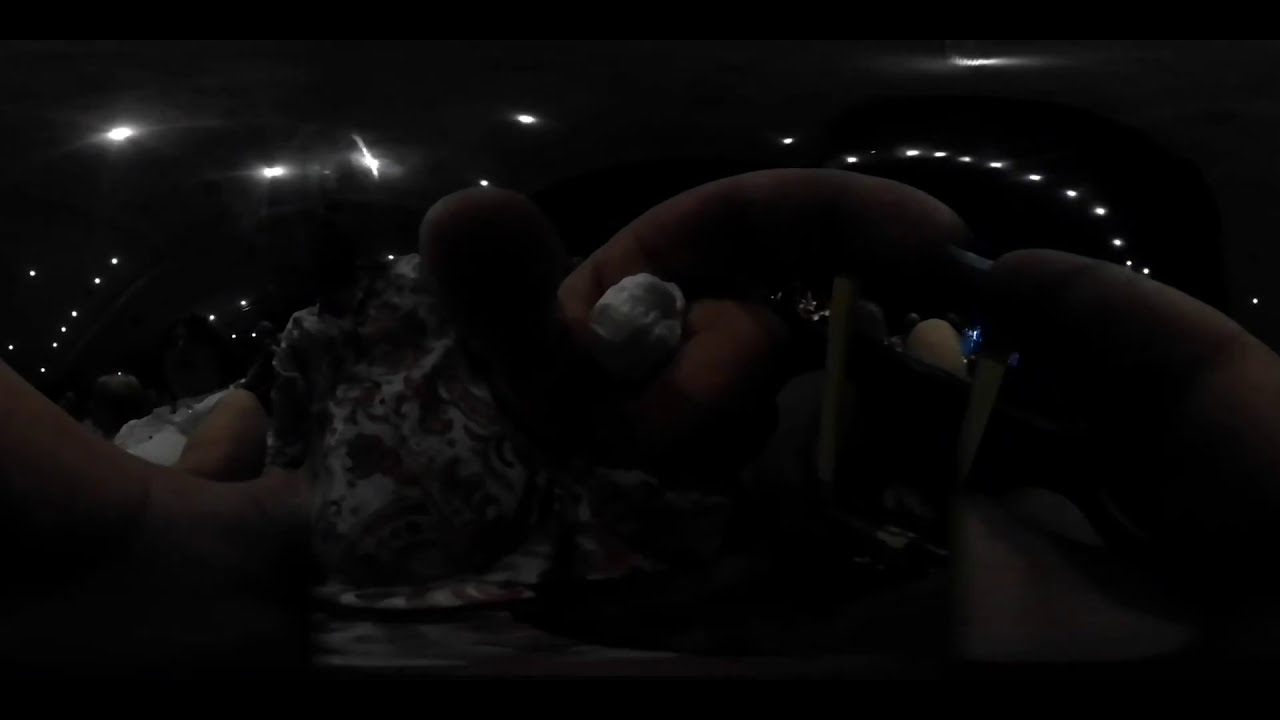This image appears to be taken using a fisheye or curved filter, leading to a somewhat unclear and distorted view. It seems the photo was clicked from inside a vehicle while passing through a dark tunnel. The darkened scene is punctuated by white lights arranged in rows on the tunnel's ceiling and floor, giving an almost ethereal glow. In the foreground, the hands of a person near the camera suggest it's a candid shot, possibly by accident. To the left, there's a person in a white sleeveless shirt sitting, though details are hazy due to the low light. The bottom of the image features horizontal black strips, which might be reflections or elements of the vehicle. The overall ambiance suggests an indoor environment characterized by a dramatic play of darkness and light.